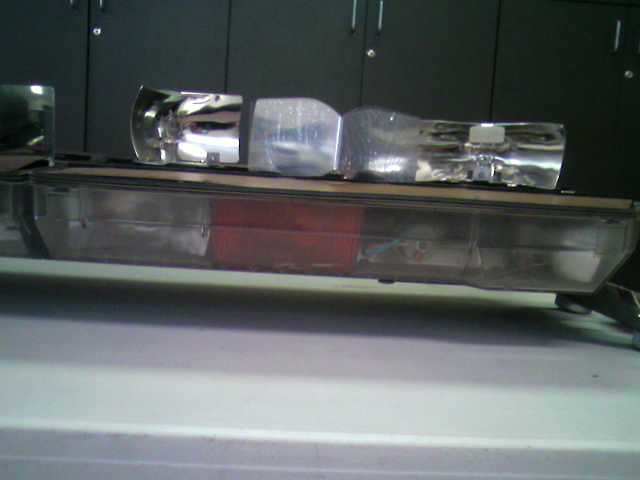This slightly out-of-focus indoor photograph centers on a vehicle-mounted set of rectangular lights, typically seen on emergency vehicles such as police cars or ambulances. The outer protective lens of one light has been removed, revealing the chrome reflectors and light bulbs within. These concave reflectors, while reflecting the unclear background image, illustrate an attempt to either inspect or replace the light bulbs.

The vehicle's roof and a white foreground—possibly a table or the floor—are visible. Resting on this white surface is a clear, raised rectangular container with visible engineering components such as wires and plastic pieces. A notable reflective, metal object similar to a satellite dish-like item sits atop this container. 

Behind this setup are dark greenish-black storage cabinets featuring small silver handles and keyholes on closed vertical doors, extending in rows. The scene is detailed yet slightly blurred, lending an enigmatic touch to the otherwise clinical environment.